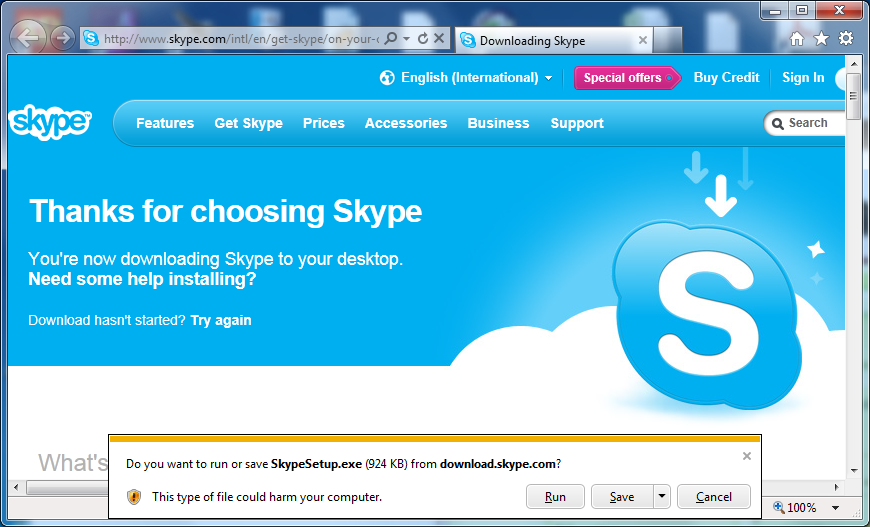Screenshot of the Skype download webpage.

The image captures a browser window displaying the official Skype download page, with the URL clearly visible in the address bar as "Skype.com". The browser tab is labeled "Downloading Skype", confirming the ongoing download process. The central section of the page features a message in large font: "Thanks for choosing Skype. You're now downloading Skype to your desktop." Below this, there are additional instructions: "Need some help installing? Download hasn't started? Try again."

On the right side of the page, the recognizable Skype logo—an "S" encased in a stylized cloud—is prominently displayed, with arrows pointing downward towards it, signifying the download process. The background features a blue and white cloud design, consistent with Skype's brand colors.

At the bottom of the screen, a pop-up notification appears, asking, "Do you want to run or save skypesetup.exe (924 KB) from download.skype.com?" This window includes a cautionary warning icon, likely from Windows Defender, alerting the user that "this type of file could harm your computer". Three action buttons are available: "Run", "Save", and "Cancel", with the "Save" button offering a drop-down menu for additional options. 

The overall blue theme and design elements reinforce Skype's distinctive interface and user experience.